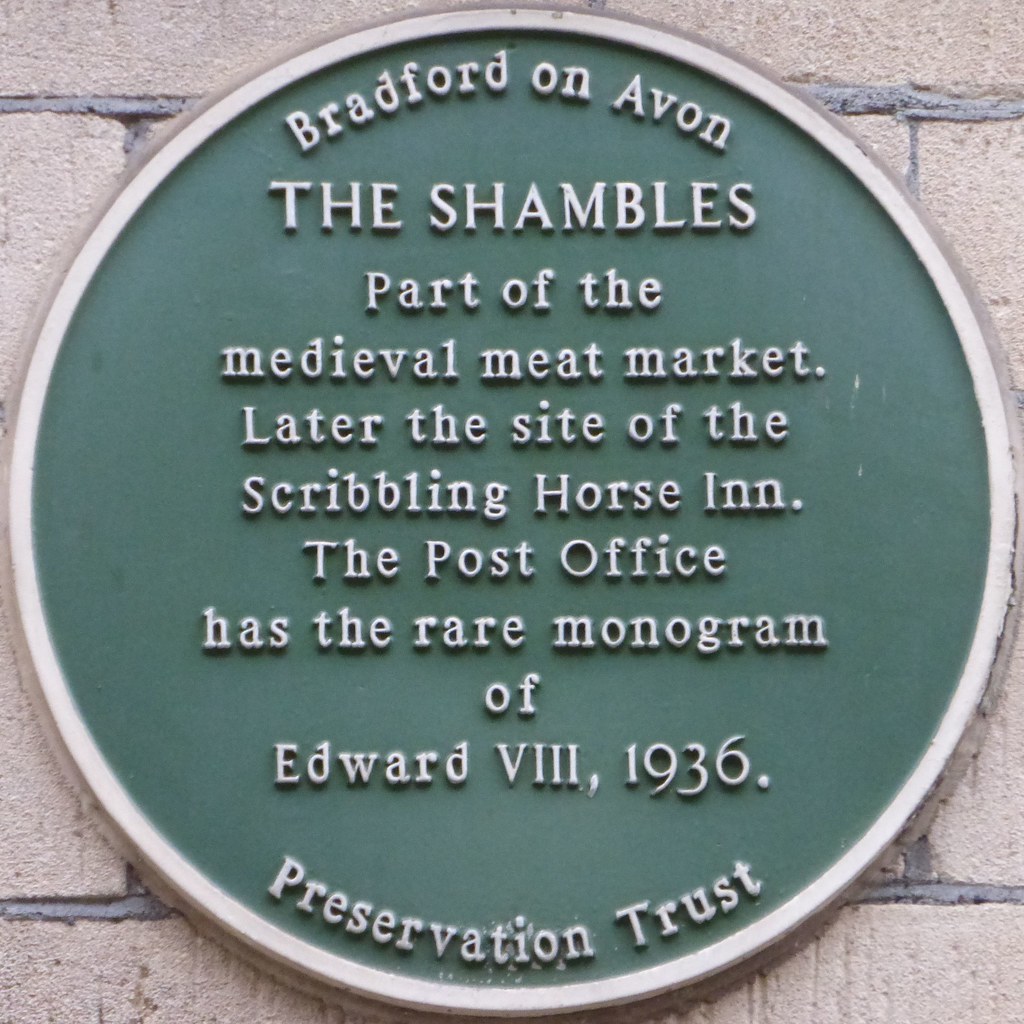The close-up photograph showcases a circular placard cemented onto a gray brick wall with black or gray mortar. The placard, painted green with a white, possibly silver, border, features blocky embossed white text. At the top, it reads, "Bradford on Avon," followed by "The Shambles" in large capital letters. Below, it describes, "Part of the Medieval Meat Market, later the site of the Scribbling Horse Inn." Additionally, the text notes, "The post office has the rare monogram of Edward VIII, 1936." Finishing at the bottom, it reads "Preservation Trust," curved along the edge.